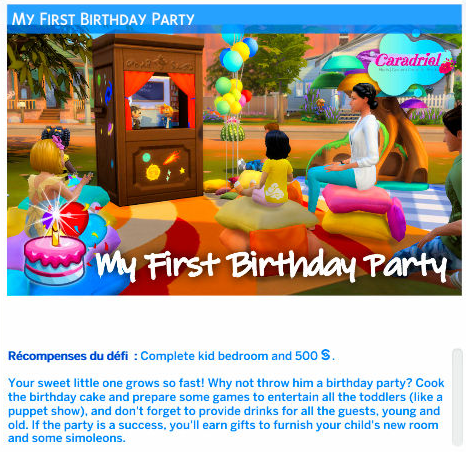This is an image from a Stuff Pack advertisement for the video game The Sims 4, showcasing the "My First Birthday Party" set. At the top and bottom of the image, a blue banner reads "My First Birthday Party." In the center of the bottom banner, an illustration of a birthday cake is prominently displayed, featuring a white cake with a pink stripe, pink frosting, and a gold candle on top. 

The scene is lively, depicting four children seated on colorful pillows atop a carpet with swirling patterns of orange, red, and white. These children are engrossed in watching an entertaining puppet show. Next to the puppet theater, a festive array of balloons in blue, yellow, green, red, and pink adds to the celebratory atmosphere.

On the right side of the image, a woman can be seen sitting comfortably on a collection of pink and yellow pillows, and behind her, another woman is seated on the ground. The bottom of the image also includes text describing the pack's contents, stating it features a complete kid's bedroom set and is priced at $500.